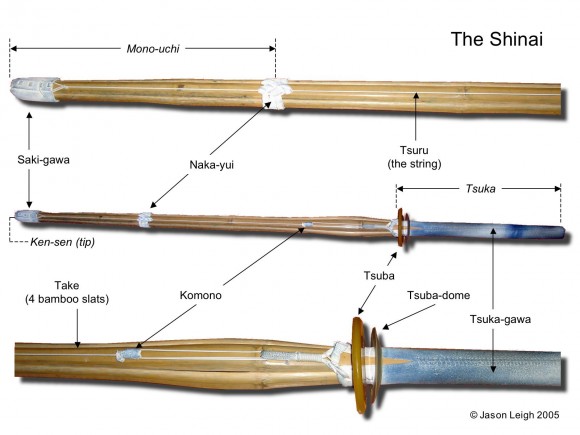This detailed infographic, titled "THE SHINAI," illustrates three different views of a traditional bamboo sword used in Kendo. The top image showcases the entire shinai, made of bamboo with a white tape wrapping in the middle and a white cover on the left end, identified as the "SAKIGAWA." An arrow points to this area labeled with the Japanese term. The middle image displays the full length of the shinai, emphasizing its light brown hilt and light blue handle, along with the same bamboo structure and white tape. The bottom image provides a close-up of the handle, hilt, and half of the bamboo blade. Key parts of the sword are highlighted with arrows and text, such as "MANO UCHI" (indicating the length between the white tape and the end), "TSURU" (with the translation "the string" in parentheses), "NAKAYUI" (pointing to the middle tape), and names for various parts like the "TAKE" (bamboo slats), "KAMONO," "SUBA," "SUBADOM," and "SUKIGAWA." The comprehensive guide is supplemented with copyright information in the bottom right corner, attributing the image to Jason Lee, 2005.